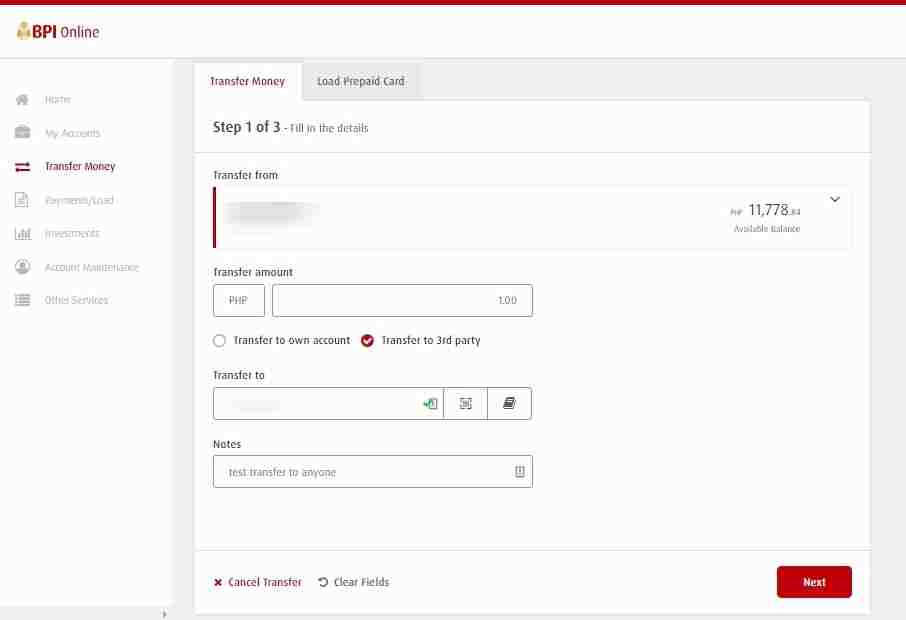Here is the cleaned-up and detailed descriptive caption for the image:

---

Screenshot of the BPI Online website in the process of transferring money. 

The interface shows "Step one of three" in the process: "Fill in the details." There is a dropdown menu next to the label "Transfer from" indicating a current balance of $11,778. Below, there's a field to enter the "Transfer amount," with a placeholder text "POP, $1." 

To specify the recipient, options include:

- "Transfer to own account" represented with an empty circle.
- "Transfer to third party" marked with a red checkmark inside a circle.
- "Transfer to" (destination unspecified) featuring a green symbol, a gray square with a dot in the center, and an icon resembling a black book.

A "Notes" section includes the text "test transfer to anyone" next to a trash can icon. 

Action buttons at the bottom offer choices to "Cancel transfer," "Clear fields," and proceed to the "Next" step.

The left sidebar menu, highlighted in red for the "Transfer Money" option, also includes links to "Home," "My Accounts," "Payment/Fraud," "Investments," "Account Administrator," and "Other Services." 

A thin red line runs along the top of the interface, while the background features a clean, white, and gray color scheme. On the bottom right, there's a prominent red button labeled "Next."

---

This revised caption provides a detailed and organized description of the screenshot, enhancing clarity for readers.